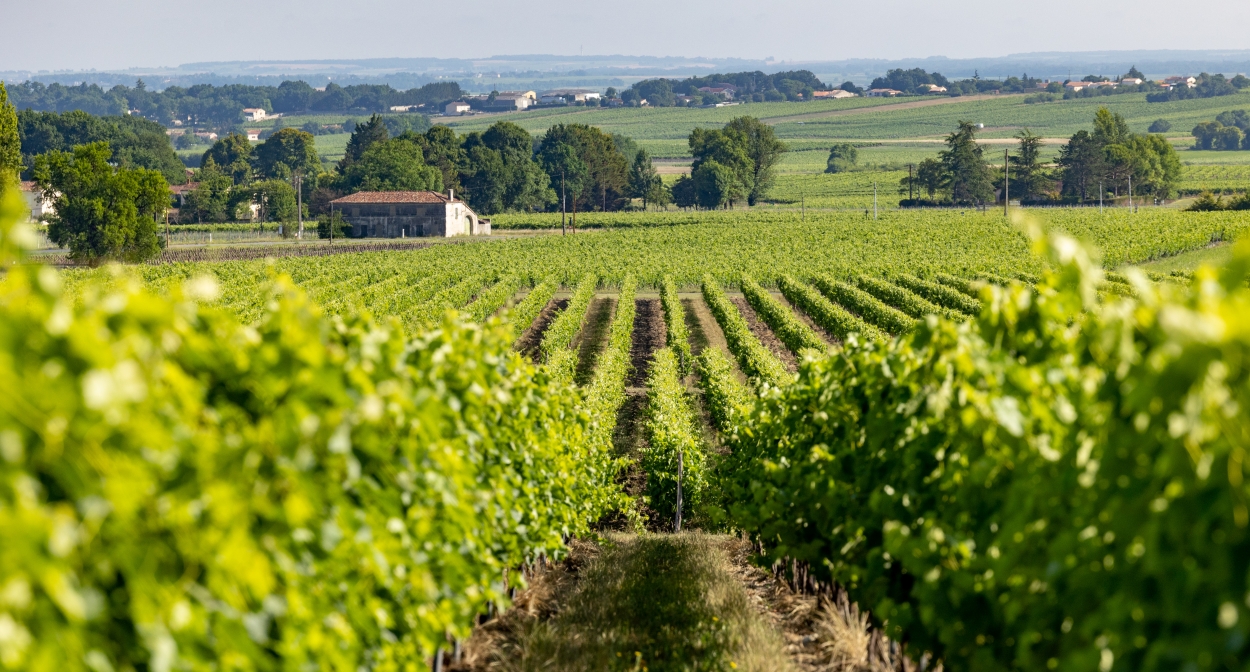The photograph showcases a picturesque rural landscape taken from the midst of a field filled with green bushes and hedges. The scene is framed by verdant crops planted in neat rows, possibly vineyard or citrus plants, with the sunlight intensifying the green hues more prominently on the left side of the field. In the foreground, short grass is visible between the rows, gradually blending into a thicker crop field further beyond. Toward the horizon, there stands a quaint, small white farmhouse with a red-tiled roof, which adds a rustic charm to the view. Behind the farmhouse, a dense cluster of trees forms a beautiful green backdrop. Further in the distance, expansive open fields stretch out, interspersed with more houses and patches of woodland, leading up to distant mountains that frame the idyllic scene under a bright, blue daytime sky.